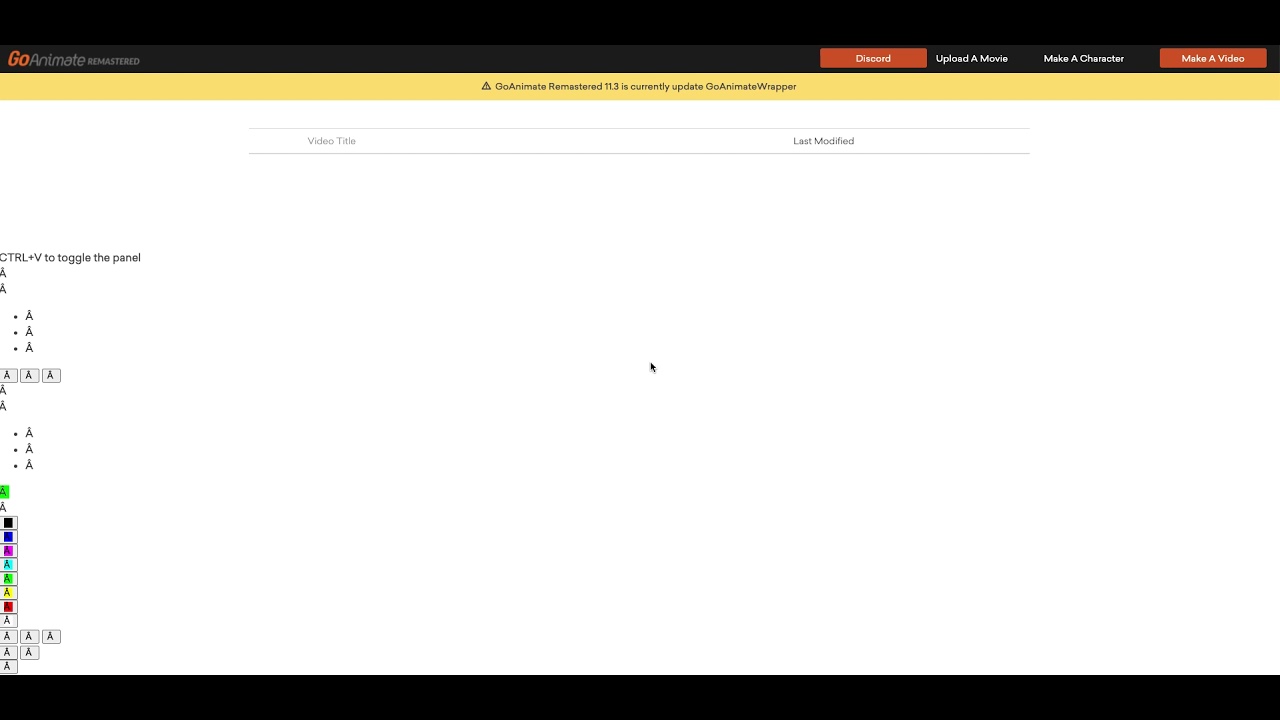Here is a detailed description of the image based on the voice caption provided:

---

The screenshot depicts an interface from the GoAnimate platform. At the very top, there is a black header featuring the words "Go Animate" followed by an unreadable word. The text "Go" is rendered in an orange font, while the rest of the text is in grey. On the far right side of the header, there are options labeled "Discord," "Upload," and "More," followed by two buttons labeled "Make a Character" and "Make a Video."

Beneath the header is a yellow subheader displaying the text "Go Animate Wrapper 11.3 is currently up-to-date" (with "Go Animals" being partially visible and assumed to be part of the title/version detail).

The main section of the screen contains a large white rectangle with a header that reads "Video Title" and "Last Modified." Along the right side of this section, there are various symbols and abbreviations, primarily denoted by the letter "A" in different formats:

- "Control + V to toggle the panel"
- Several "A" symbols, some with dots preceding them (e.g., ".A .A .A"), continuing downwards.
- A green square with a plus symbol.
- A black square with a plus symbol.
- A blue square, a magenta square.
- An "A" in a turquoise square.
- An "A" in a green square.
- An "A" in a cream-colored square.
- A burgundy square, followed by:
    - A single "A"
    - Three "A"s vertically.
    - Two "A"s vertically.
    - A single "A"
 
The image concludes with a black footer.

---

This detailed description captures the visual elements and arrangement of the given image.